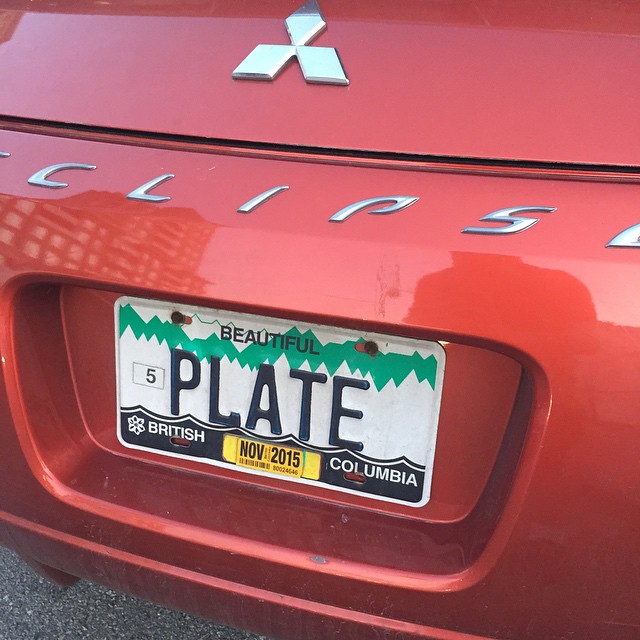This color photograph, presented in a square format, captures the back end of a Mitsubishi Eclipse in a vibrant candy apple red or blood orange hue. The setting appears to be outdoors, evidenced by a slight part of the surrounding area visible in the bottom left corner, revealing an asphalt or concrete surface. The focal point is the vehicle's rear, showcasing the Mitsubishi logo prominently at the top, with the partially visible word "Eclipse" beneath it. The license plate, set against a yellow background with black text, reads "beautiful" in smaller text and "plate 5" in larger text, with identifiers for "British Columbia" and a tag indicating "November 2015" on it. Additionally, there are green zigzag lines at the top of the plate. The car's reflective surface captures a faint image of a building and an indistinct figure, likely the photographer. The tight framing excludes views of the windows or wheels, emphasizing the car's branding and plate details.